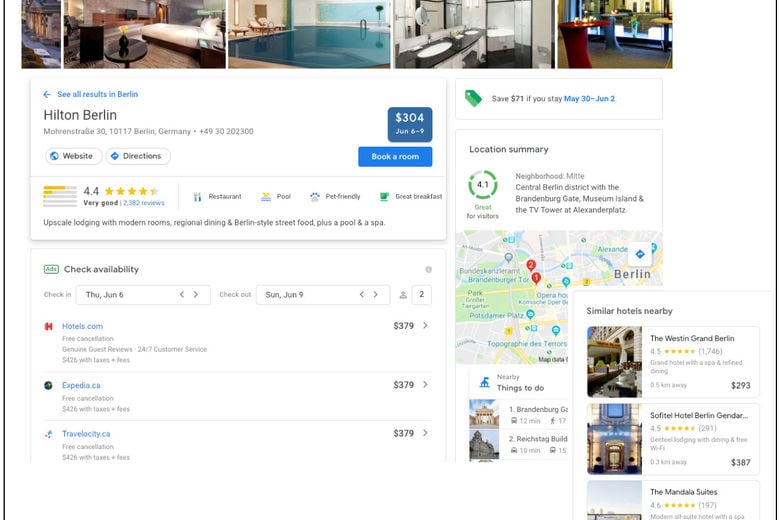This screenshot captures a detailed Google search results page for the Hilton Berlin Hotel. At the top, there are several images showcasing various amenities of the hotel, including a well-made bed, a pristine pool, a modern bathroom, and a vibrant restaurant or bar area.

Directly below the images, there's a navigation text link in blue that allows users to return to viewing all hotel results in Berlin. It appears the user has selected "Hilton Berlin," which is stated in bold black text, with the hotel's address listed just beneath. The address mentions Berlin, Germany, accompanied by a phone number, which is not fully detailed here. 

On the right-hand side, there is a conspicuous blue button displaying the pricing and availability for the dates June 6th to June 9th, quoted at $304. There's another blue button below offering an option to book a room. Adjacent to the hotel name, two additional buttons provide links to the hotel’s website and directions.

Further down, the hotel is reviewed with an aggregate rating of 4.4 stars out of 5, based on 2,382 reviews, indicating a "Very Good" status. There are highlighted icons for amenities, including a restaurant, pool, pet-friendly facilities, and great breakfast options. The description elaborates that this upscale lodging features modern rooms, regional dining experiences, Berlin-style street food, a pool, and a spa.

The section below this provides an availability check with the specified check-in date of Thursday, June 6th, and check-out date of Sunday, June 9th. Users can adjust these dates and the number of guests, which is currently set to two. Prices from three different booking websites—Hotels.com, Expedia.ca, and Travel Velocity.ca—are each listed at $379.

On the right-hand side, there is a special offer text box mentioning a $71 saving for stays between May 30th and June 2nd. Below this offer, there is a location summary for the Mitte district, central Berlin, highlighting notable attractions such as the Brandenburg Gate, Museum Island, and the TV Tower. A map provides a visual for nearby attractions.

Additionally, a text box appears at the end, indicating similar nearby hotels, offering alternative lodging options with three suggestions listed.